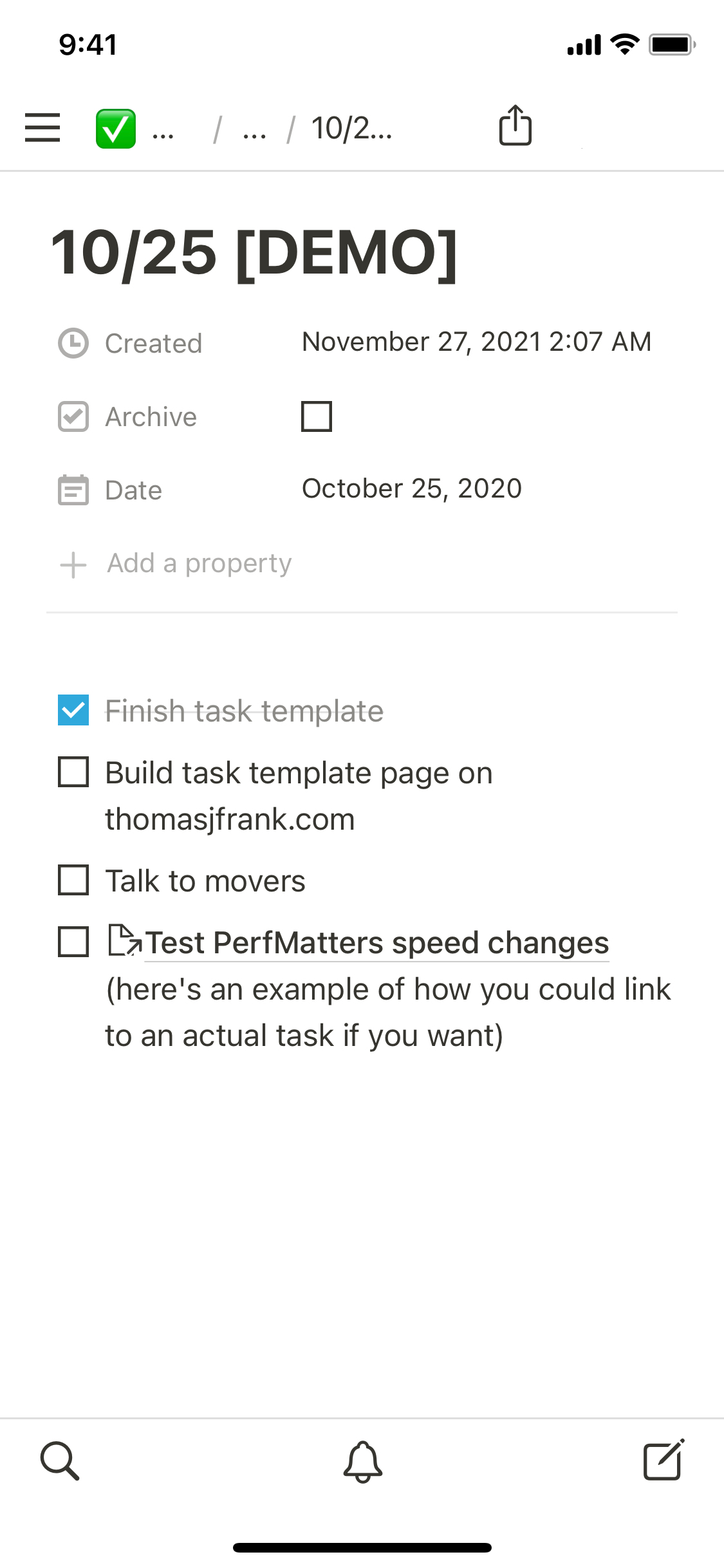Image Caption: 

The image is a detailed screenshot of a task management app or platform, likely taken on a mobile device as indicated by the top-left timestamp displaying "9:41 AM." The background is white, and various symbols and illustrative text elements are organized in a structured manner.

At the top, there's a green checkbox with a white checkmark signifying a completed task. This is followed by a series of ellipses and slashes (".../.../10/2..."). Below this sequence, there is an icon of a box with an arrow pointing upwards, indicating an export or upload option.

Further down, there is a bold text line reading "Texas," followed by the date "10/25" within brackets labeled as "Demo." Under this is an icon of a small clock, accompanied by the timestamp "Created: November 27th, 2021 2:07 AM." 

Following the timestamp, there are several other components:
- A checkbox with the label "Archive" next to it, which is not checked.
- A calendar icon with the date "October 25th, 2020" beside it.
- A plus symbol leading to an option labeled "Add a Property" in light gray text.

Below these elements is a sequence of checkboxes with respective labels:
- A blue checkbox with a white checkmark labeled "Finish tasks template."
- Several unchecked boxes with respective tasks next to them, including: 
  - "Build task template page on ThomasJFrank.com"
  - "Talk to movers"
  - "Test performance matters speed changes"
  (This section includes a note indicating how to link to an actual task in parentheses.)

At the very bottom of the image, there is a horizontal line followed by a cluster of icons, including a magnifying glass (likely for search), a bell (for notifications), and a pen-and-pad symbol (probably for notes or writing).

The entire image displays a clean and organized layout typical of task management or to-do list apps, capturing various aspects of task organization and scheduling.